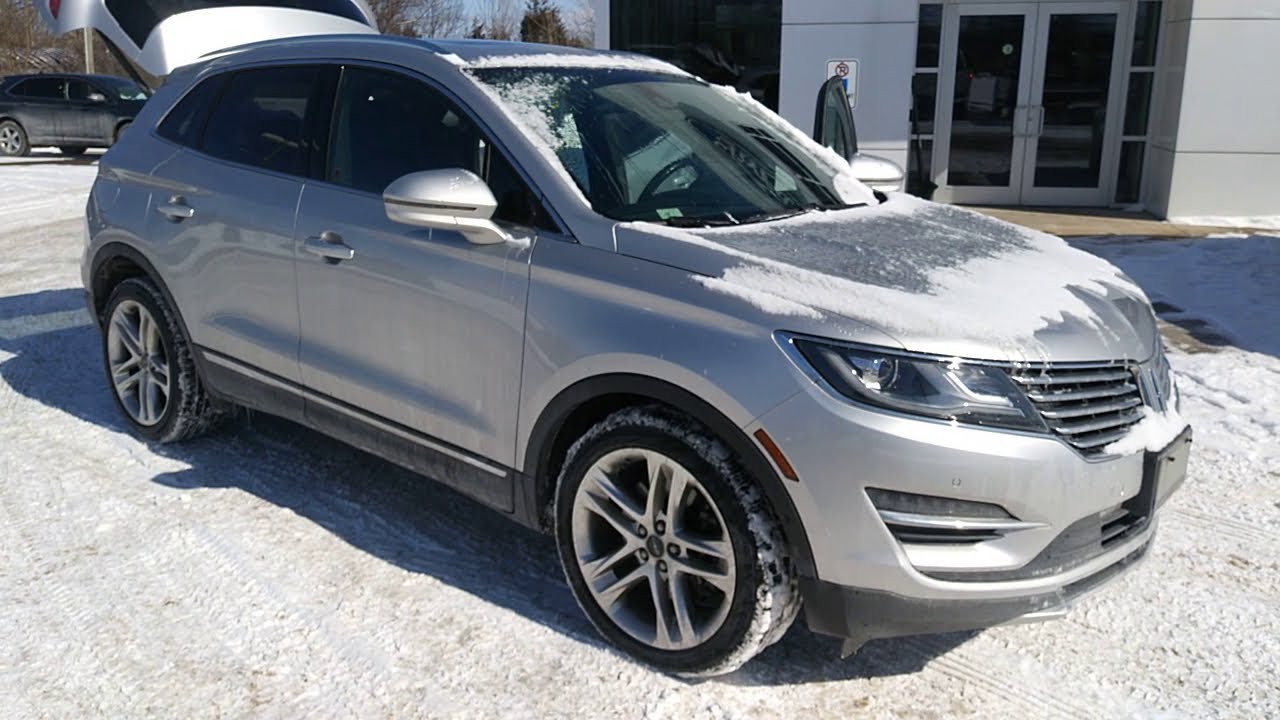This detailed photo captures a silver four-door crossover vehicle, possibly a Subaru Outback, prominently positioned at a diagonal angle, facing right in a horizontal rectangular frame. The crossover is coated with snow residue—mainly on the hood, front license plate, and windshield, with additional traces on the tires. The snow appears to be melting in the bright, sunny daytime setting. The driver's side door and the trunk are both open, and the windows are tinted.

The car is parked on what seems to be a gravel surface, though it could be packed snow. The backdrop features a building with silver paneled walls and tinted two-door entrances. In the distance, towards the top left of the image, another dark-colored SUV is visible. Additionally, there appears to be a small body of water, resembling a pond, located towards the right corner of the image. The entire composition suggests a clean, brisk outdoor environment, possibly near a car showroom or similar structure.